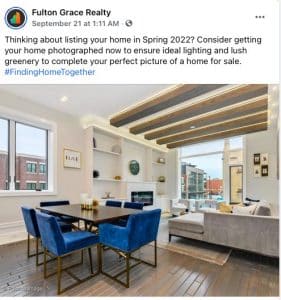This image shows a social media post by Fulton Grace Realty, with its logo displayed on a small circular graphic against a black background at the top. The post is dated September 21st at 1:11 a.m. To the right, there are three horizontally aligned dots indicating further options. The main text of the post reads, "Thinking about listing your home in spring 2022? Consider getting your home photographed now to ensure ideal lighting and lush greenery to complete your perfect picture of a home for sale." Below the text, in blue font, is the hashtag "#FindingHomeTogether."

The post also includes an image of an open floor concept interior. The space features a white ceiling and warmly painted walls. The kitchen area has two windows that allow natural light to flood in. Adjacent to the kitchen is a dining area with a table surrounded by six blue chairs. The living room, located within the same open space, showcases a comfortable couch with a chaise lounge, complemented by a cozy area rug. The room also features a TV, several pictures on the wall, and elegant vases as decorations. A large picture window offers a scenic view, and a balcony can be seen with two additional chairs, suggesting an inviting spot for relaxation.